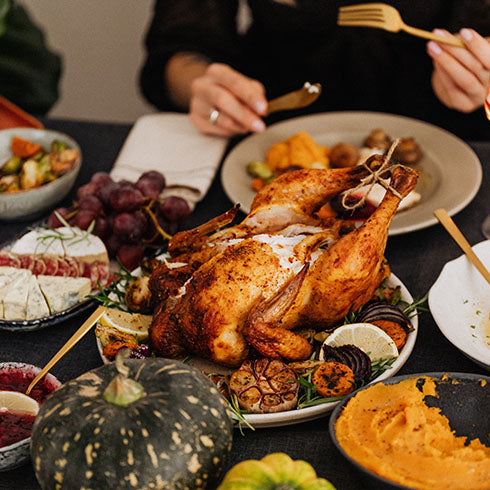The photograph captures a beautifully arranged Thanksgiving dinner from a top-down perspective. At the center of the image, on a charcoal gray tablecloth, sits a plump roasted turkey on a round white platter. The turkey is surrounded by garnishes of grilled lemons, grilled onions, and rosemary sprigs. To the front of the composition, there are two gourds—one variegated green and white, and the other yellow. To the right of the turkey, a bowl of mashed sweet potatoes is half-empty, suggesting an ongoing meal. Additionally, on the left, a bowl of cranberry relish with a lemon slice and a golden spoon can be seen, adding a pop of color.

In the background, a person in a black sweater is visible, holding a golden knife and fork with painted nails and a ring on their hand, emphasizing a female presence. The person's plate is filled with food, highlighting the action of dining. Surrounding the turkey are various appetizers, including a cheese plate with blue cheese, salami slices, and red grapes, as well as a bowl of Brussels sprouts. The color palette of the spread features warm fall hues: greens, oranges, browns, muted reds, bright orange sweet potatoes, and the deep red of the grapes, enhancing the seasonal feel of this Thanksgiving feast. The entire scene oozes the essence of a cozy, festive fall meal in progress.